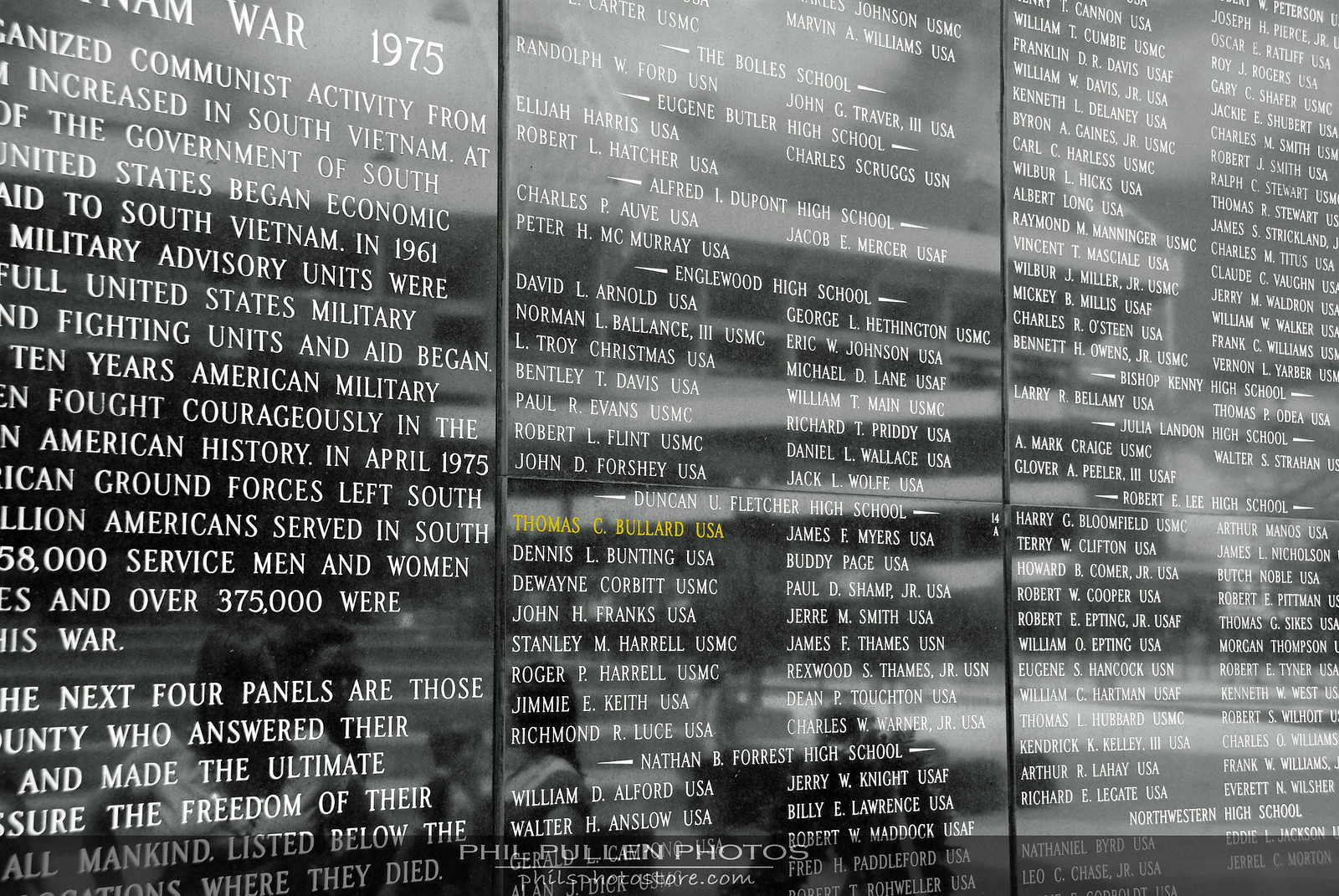This detailed image depicts a solemn memorial dedicated to the Vietnam War, specifically referencing the year 1975. The memorial wall, constructed of black granite panels resembling tombstones, features an extensive list of names etched in white letters. These names are organized under various titles, including notable mentions of educational institutions such as the Bolles School, Eugene Butler High School, Alfred I. DuPont High School, and Englewood High School. Each name is accompanied by the military branch of the individual, such as USN (United States Navy) and USA (United States Army).

Positioned on the far left of the wall is a speech providing a fragmented but poignant description of the Vietnam War. Phrases visible in the text mention "communist activity," "South Vietnam," and "military advisory units," offering insight into the historical context and U.S. involvement in the conflict beginning in 1961. The wall stands upright, evoking the presence of a tombstone, and the setting suggests it is part of an outdoor memorial structure, likely visited during solemn events to honor the fallen. The sheer number of names, coupled with the gravitas of the memorial's design, makes the experience of viewing it overwhelmingly moving.